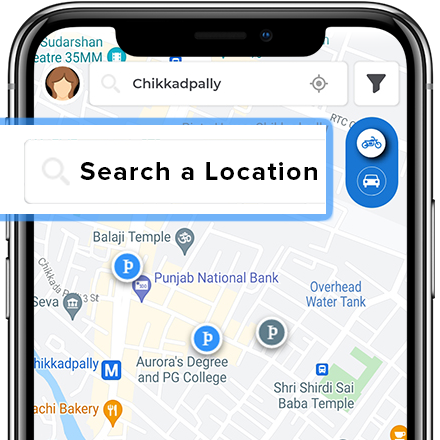This image is a screenshot taken from someone's phone screen. At the top, the screen displays the location name "Chickapally" in bold text. Below this, there is a prominent rectangular search bar with a faint magnifying glass icon on the left side, housed within a white background. This search bar is outlined in a bluish color, which extends across the top and right side, down to the bottom, but not the left side, possibly due to the screen's cutoff.

Just below the search bar, there is a small, cartoon-style profile picture of a person. The profile picture shows only the top part of the person's head with hair, and the face is featureless, lacking eyes, nose, and mouth.

As you scroll further down the screen, various place names are listed. These include Balajai Temple, Punjab National Bank, Aurora's Degree and PG College, Shree Shrard Shai Baba Temple, and Overhead Water Tank. Each of these names appears in distinct text, indicating landmarks or points of interest in the Chickapally area.